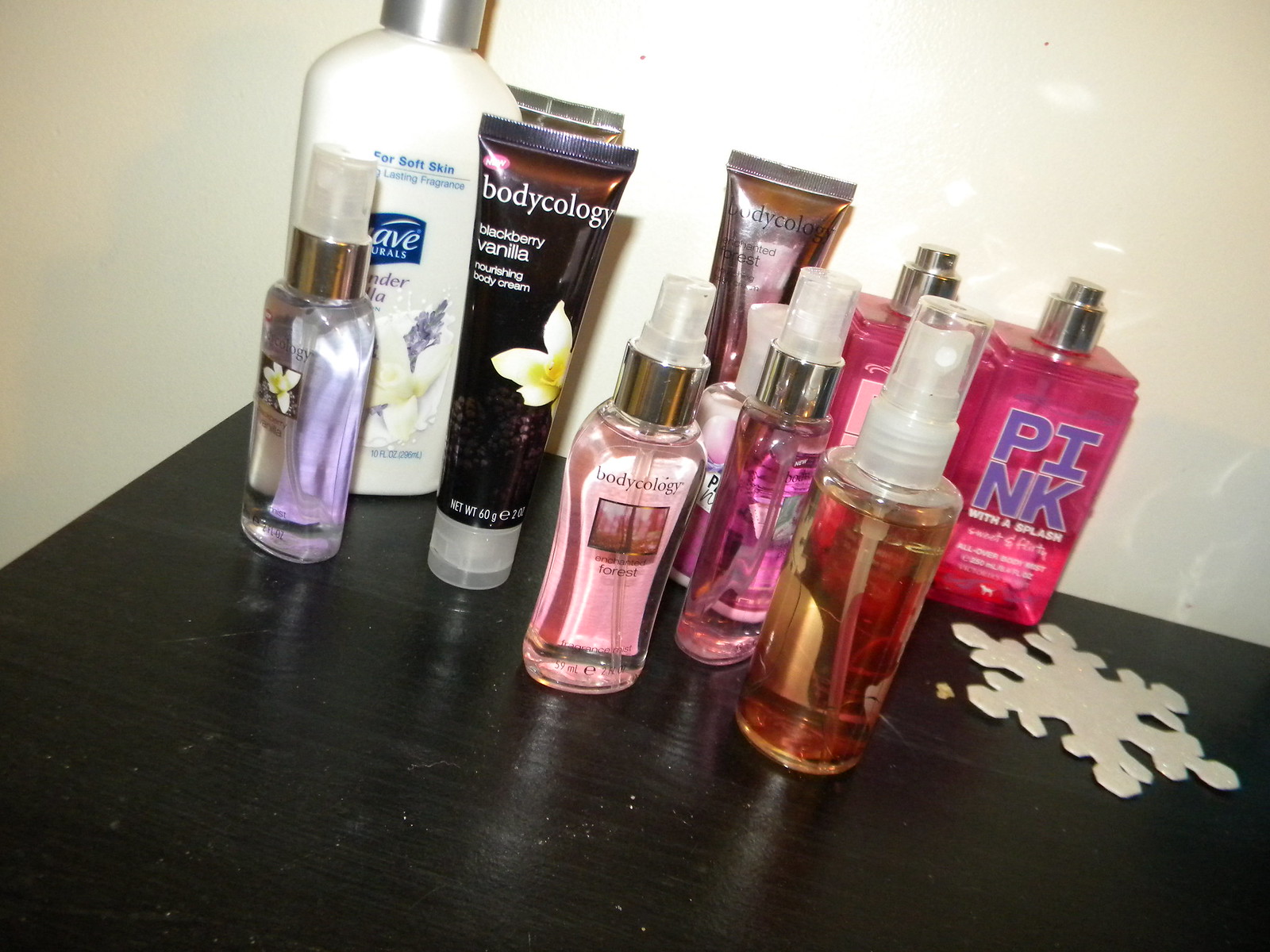This is an angled, brightly-lit photograph—likely taken with a flash—that showcases a collection of ten women's toiletry and cosmetic products, arranged on a dark, possibly black, wooden table surface. Dominating the scene are various bottles and tubes, including a Suave moisturizer in a white container marked for soft skin, positioned towards the back. A standout element is a flat, glittery white snowflake-shaped cutout, placed adjacent to the products on the right side of the image. Among the diverse array of items, several are identified as Bodycology products, including an upright tube of Blackberry Vanilla Nourishing Body Cream. The collection also features an assortment of body sprays in varied colors—one pink, one purple, and another with a label in all caps that spells "PINK," divided between PI in blue and NK in lavender. Each item varies in shape and size, with some bottles being cylindrical and others more distinctly shaped, some having caps while others expose their dispensers.